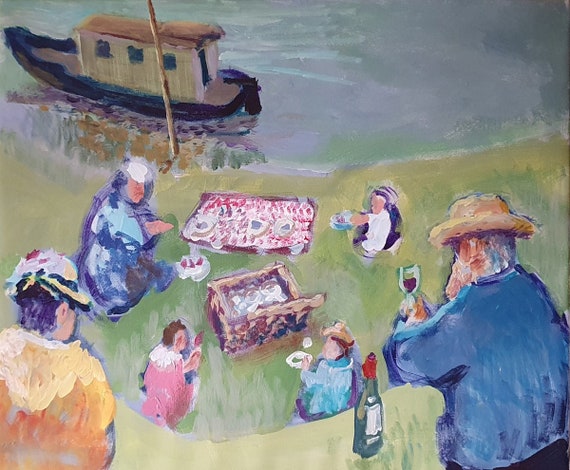This is an acrylic painting depicting a serene riverside picnic scene. In the upper left corner, there's a small tan-colored boat with a brown roof and black trim, partially in the water. The boat features a small house-like structure, a wood post or tree, and a small engine submerged in the water. Surrounding the boat is a grassy riverbank leading to a family enjoying a picnic. The picnic setup includes a red blanket, an open basket, plates, and scattered food. The people, painted with splotchy strokes, lack detailed features but convey a tranquil atmosphere. A woman with an orange-brown jacket and a white hat is seen from behind in the bottom left corner. In the far right, a man in a beige hat and blue shirt holds a half-full wine glass, with a bottle of wine bearing a red top beside him. Near him, a young girl in a pink dress with a white collar gazes up, and another child and woman are part of the picnic group, enjoying their meal together.